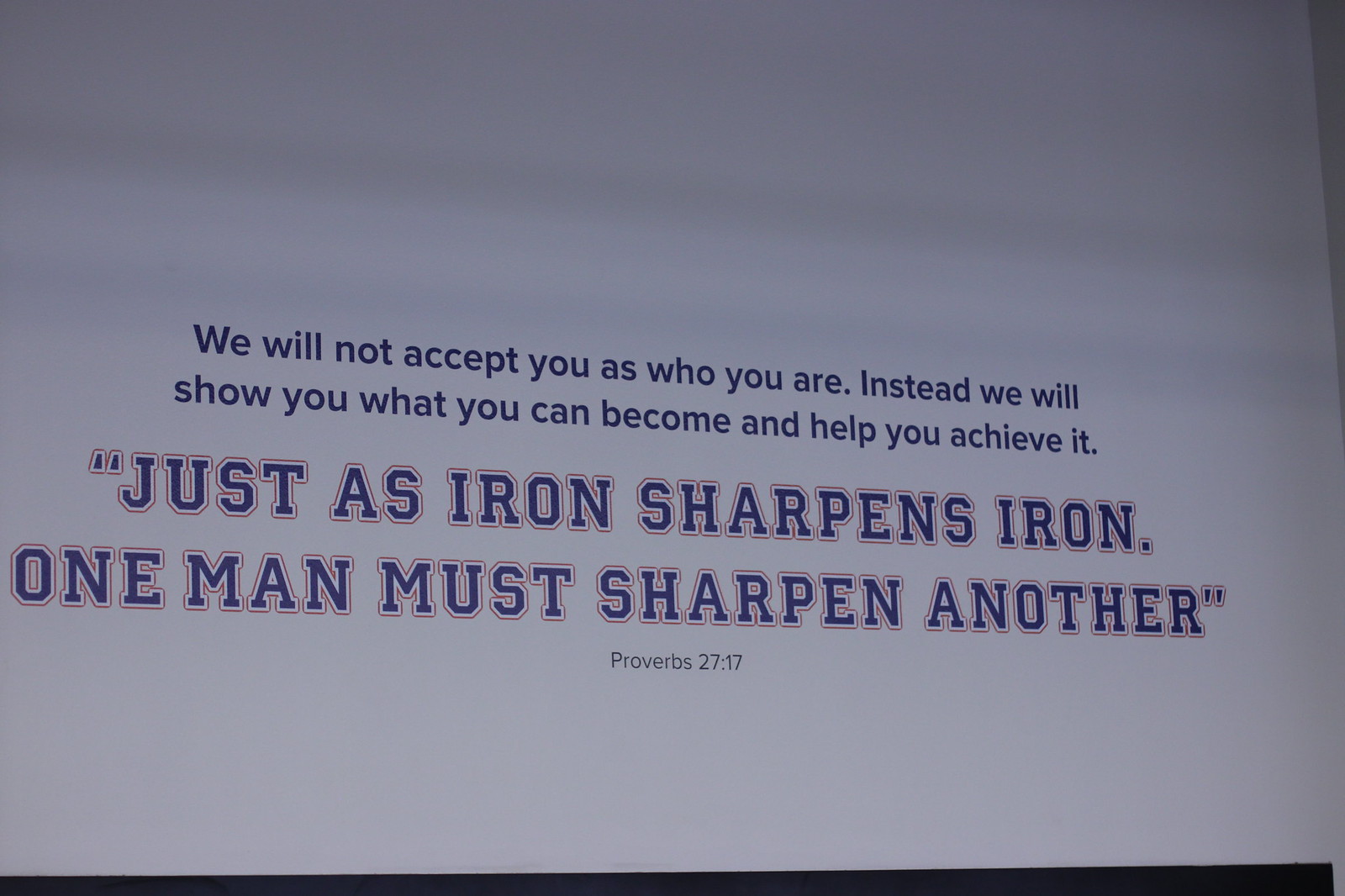The image appears to depict a motivational poster, possibly seen at a presentation or conference, with a clean white background. The text, which occupies the central portion of the image, is strategically designed across four lines with varying sizes and colors, adding depth and emphasis. The smallest text at the top states, "We will not accept you as who you are. Instead, we will show you what you can become and help you achieve it." Following this, larger, bolded text with orange outlines and quotation marks reads, "Just as iron sharpens iron, one man must sharpen another." Below this, in tiny black text, is the Bible verse reference, "Proverbs 27:17." The overall style of the poster suggests it could be something displayed in a school, sports stadium, or similar setting aimed at motivating and inspiring individuals.